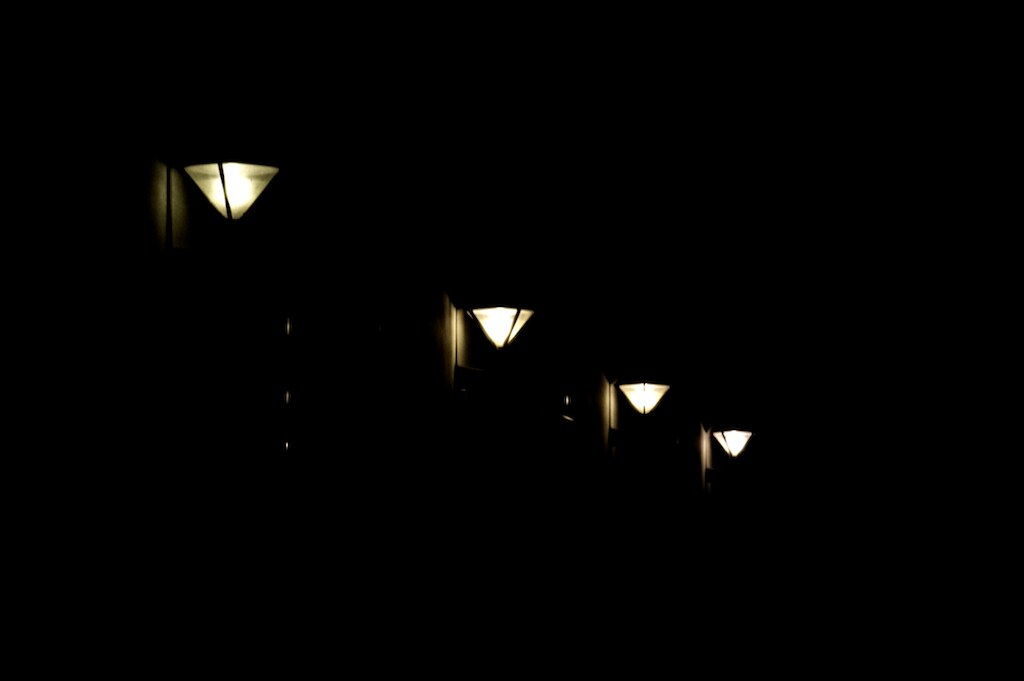The image captures a pitch-black night scene featuring four lights that emit a yellowish hue, arranged in a distinctive upside-down triangle formation. These lights, likely resembling streetlights, are staggered in distance, with one closer to the viewer and the others trailing off into the darkness. The illumination from the lights does not fully light up the area, only casting faint shadows on what appears to be a wall or similar structure, subtly hinting at a surrounding framework that supports the lights. Despite the near-total darkness of the image, the glowing bulbs create a minimal yet intriguing contrast, drawing the eye towards the sparse, gentle light they project.